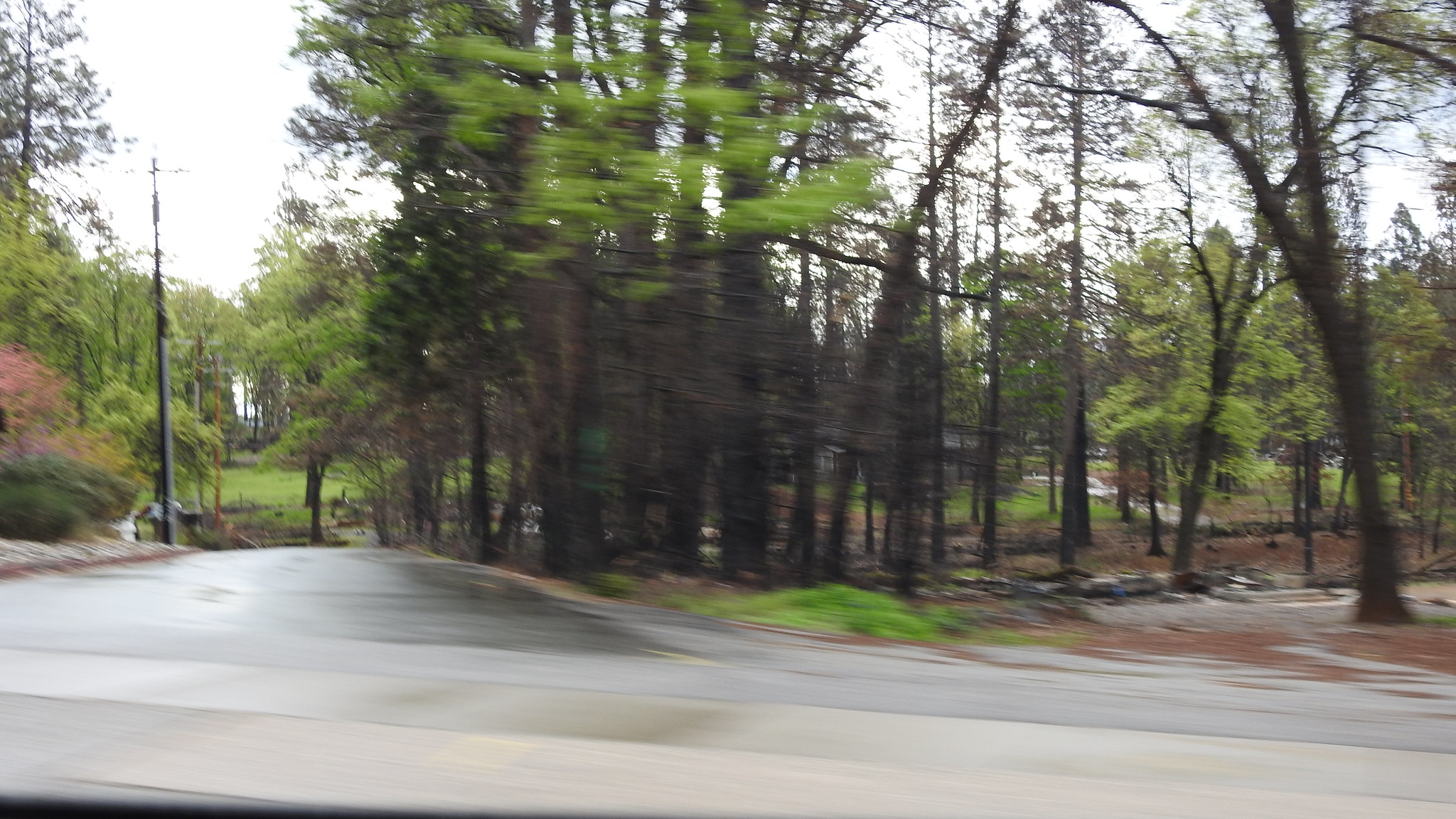This is a blurred photograph most likely taken from a moving vehicle on an overcast, rainy day. The image captures a rural street scene with a wet, tarred road that splits into a V-shape; one direction slopes downhill to the left. The center of the image is dominated by a dense cluster of trees, including dark, almost black-barked pine trees intertwined with bright green and dark green foliage. The left side of the image features another side street, leading to a scene with beautiful red and orange-leaved shrubs, pine trees, power cables on poles, and an open green field with a small building partially visible among the trees. On the right side, there’s a less densely packed area with trees having green leaves and a brown ground covered with old pine needles, interspersed with patches of bright green grass. The overall mood indicates recent rainfall, contributing to the wet appearance of the upper road, while the lower road, curving into the distance to the right, seems drier with scattered pine needles. In the V-shaped middle area where the roads meet, there is an abundance of grass and trees, some small boulders, and even hints of a home visible beyond the trees on the opposite side of the road.